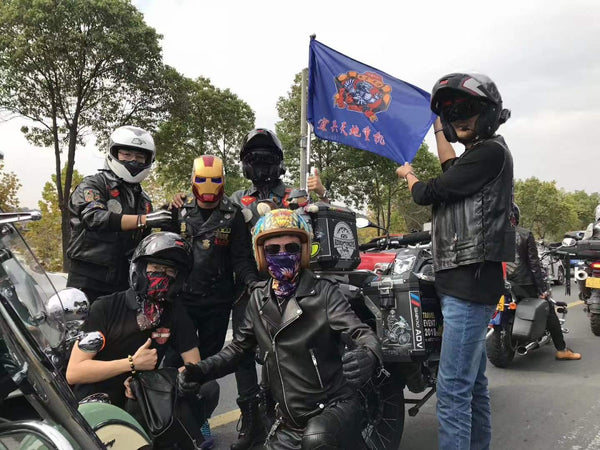This image captures a group of men, seemingly a motorcycle gang or biking crew, gathered outdoors on an overcast day. They are positioned for a group photo on a street lined with motorcycles and trees. Most of them are dressed in black leather jackets and blue jeans. The group includes a few members with distinctive helmets, including one wearing an Ironman mask and another with a Darth Vader-like helmet. A blue flag with red Asian, possibly Japanese or Chinese, characters and a complex orange and red logo is being held open by a member on the far right, who is also donning a black vest and jeans. The men exhibit a mix of standing and seated poses, with two kneeling in front— one biker in full leather attire giving a double thumbs-up, and another in a short sleeve black shirt and a bandana mask. The scene is set against a backdrop of parked motorcycles, cars, and a cloudy sky, indicating this could be a motorcycle or biker convention or a parade gathering.